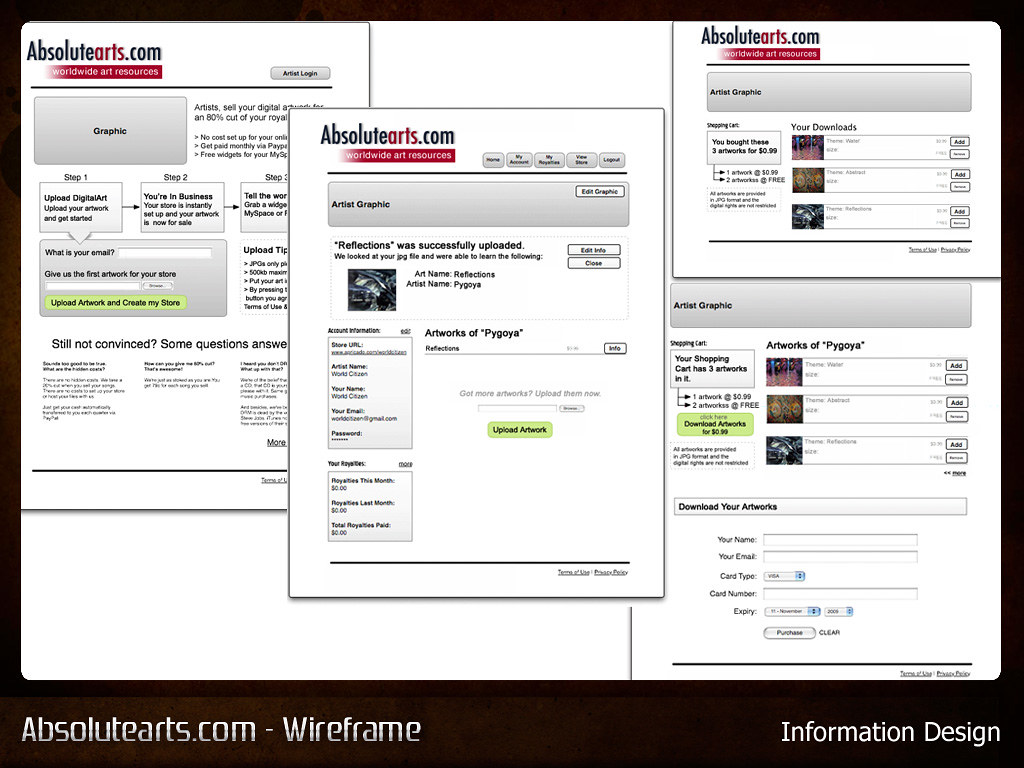The image depicts a screen capture of a website, with multiple overlapping sections suggesting different steps in an art store website builder. The primary website is identified as absolutearts.com, indicated prominently at the top left, accompanied by the tagline "Worldwide Art Resources." Below, the top left section hints at a navigation structure with tabs for user inputs such as email and artwork details. The central portion of the image provides options for uploading artwork, with further instructions on how to start setting up an art store. To the top right, there’s a visible indication of purchases, listing three art pieces bought for 99 cents each, and mentioning an artist named Pai Goya. 

The image structure is surrounded by a dark frame, thickest at the bottom, where "absolutearts.com-wireframe" and "information design" are marked in white text at the bottom left and right respectively. A notable red bar with white text runs below the website name, adding to the branding theme but remains unreadable due to its small font size. Different sections are variably sized and overlaid; the largest on the left describes initial steps including an FAQ section, while the middle section focuses on uploading graphics. The right sections display download information and shopping cart contents, visually reinforcing the website’s function as a user-centric art store builder interface.